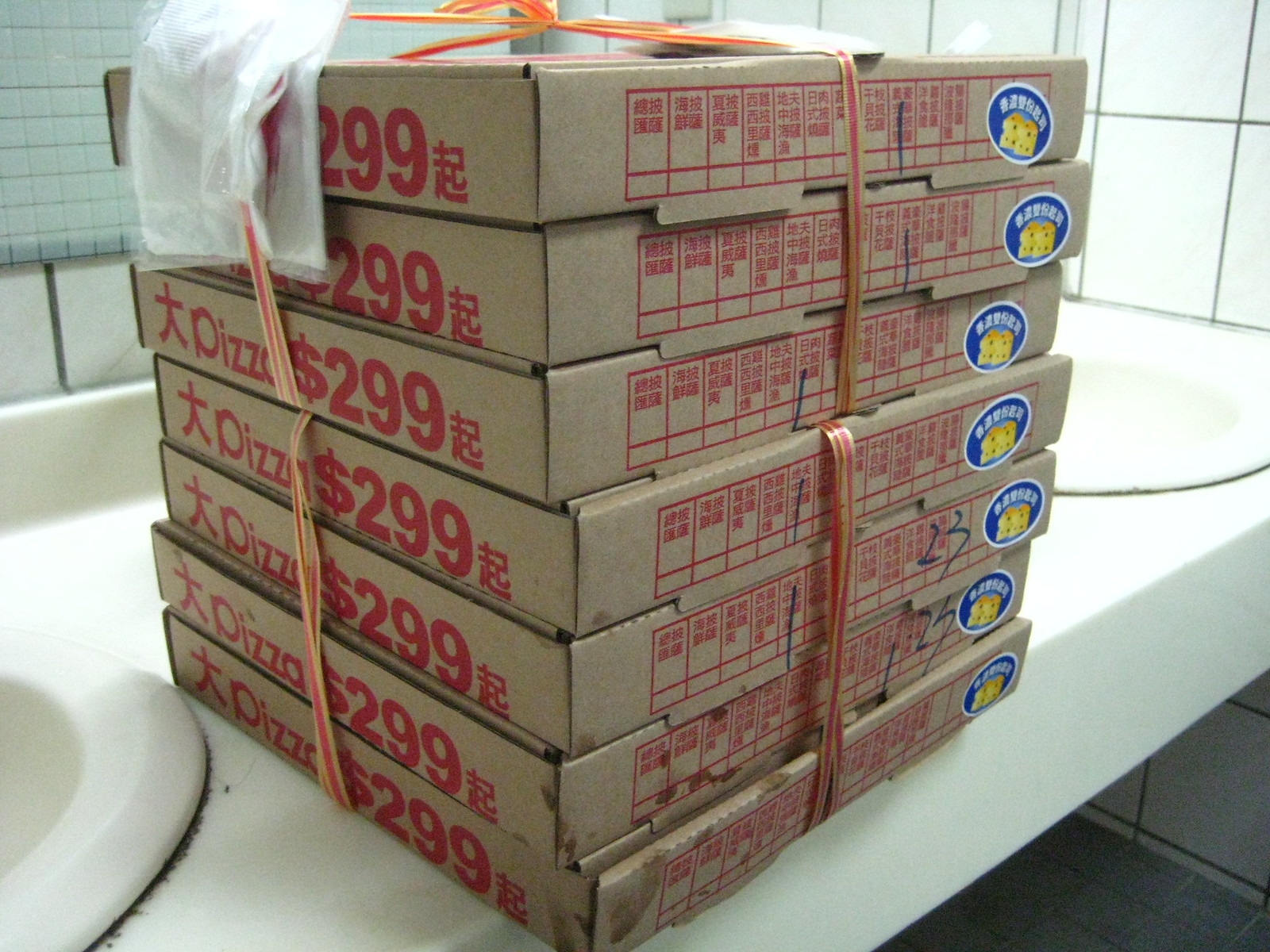In this image, there are seven pizza boxes stacked on a white bathroom counter with a sink on either side, surrounded by white tile walls. The pizza boxes, which are plain cardboard with red print, are tied together with an orange and gold ribbon. A blue and yellow sticker featuring a yellow face, possibly a cheese icon, is affixed to the left side of the boxes. Additionally, on the left side of the boxes, there is text that reads "pizza $299." There's also a reddish square chart with some writing on the right side of the boxes. Each box is marked with a blue marker, indicating possibly the type of pizza toppings, with some boxes showing specific numbers like 23 and 27. The counter appears to have some mold around the sinks, making the placement of the food boxes less appealing.